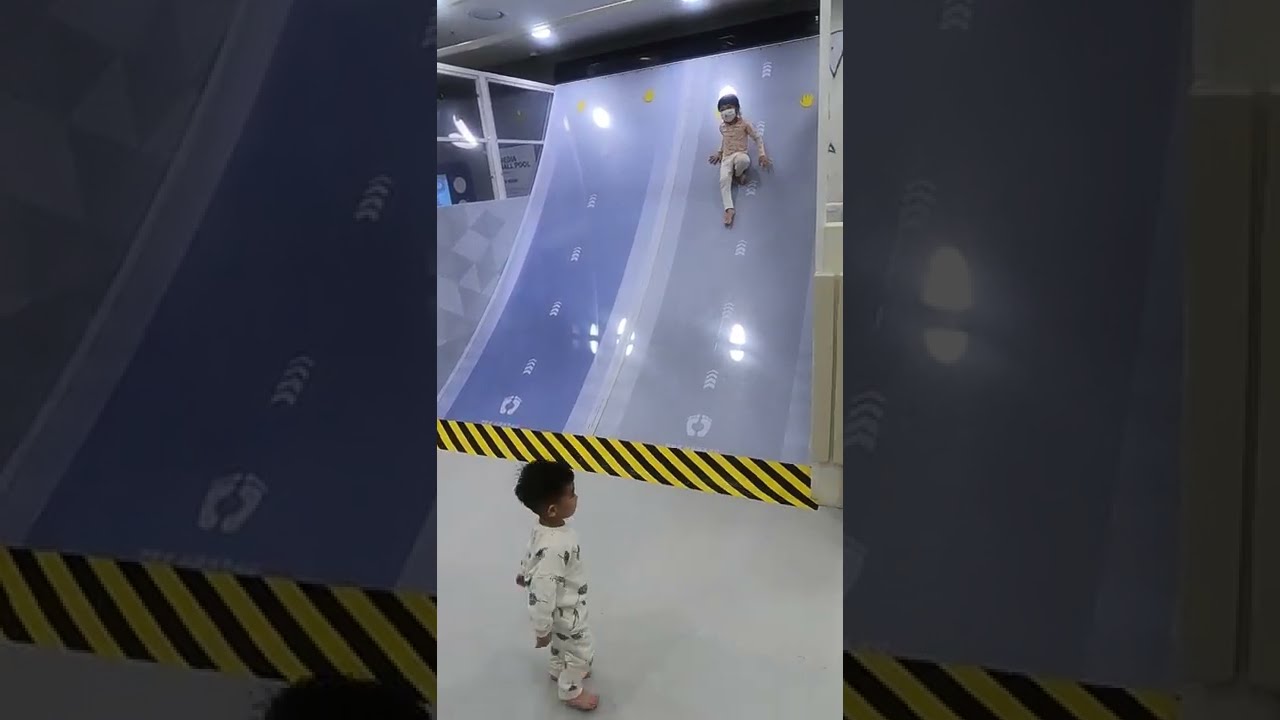The image captures an indoor play area featuring a large, steep, metallic slide, centrally positioned at an angle. The slide extends upwards around 20 to 25 feet and is adorned with diagonal black and yellow caution stripes at its base, signaling safety precautions. Descending the slide is a child, approximately a third of the way down, dressed in white pants and wearing a mask. Another child, a young boy with short brown hair, stands at the bottom of the slide, clad in an outfit that appears all white and gray. The indoor environment is illuminated by overhead spotlights. Surrounding the slide, there are cement structures to both the left and right sides of the image. The overall color palette includes shades of gray, light gray, yellow, black, tan, and silver, creating a somewhat industrial yet playful atmosphere.